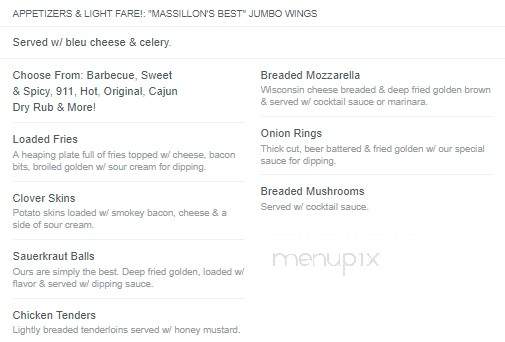#### Menu Items

**Advertisers**  
N-Light Affair's "Massillon's Best" Jumbo Wings  
*Served with Bleu Cheese & Celery*

**Choose From:**
- Barbecue
- Sweet and Spicy
- 911 Hot
- Original
- Cajun
- Cajun Dry Rub
- Warm!

**Breaded Mozzarella**  
Wisconsin Cheese, Breaded and Deep Fried to Golden Brown. Served with Cocktail Sauce and Marinara.

**Loaded Fries**  
A heaping plateful of fries, topped with cheese and bacon bits. Served golden with sour cream for dipping.

**Onion Rings**  
Thick-cut beer-battered onions, fried to golden perfection. Served with our special dipping sauce.

**Potato Skins**  
Loaded with smoky bacon and cheese, served with a side of sour cream.

**Breaded Mushrooms**  
Served with cocktail sauce.

**Sauerkraut Balls**

**Chicken Tender**  
Slightly breaded tenderloin served with honey mustard.